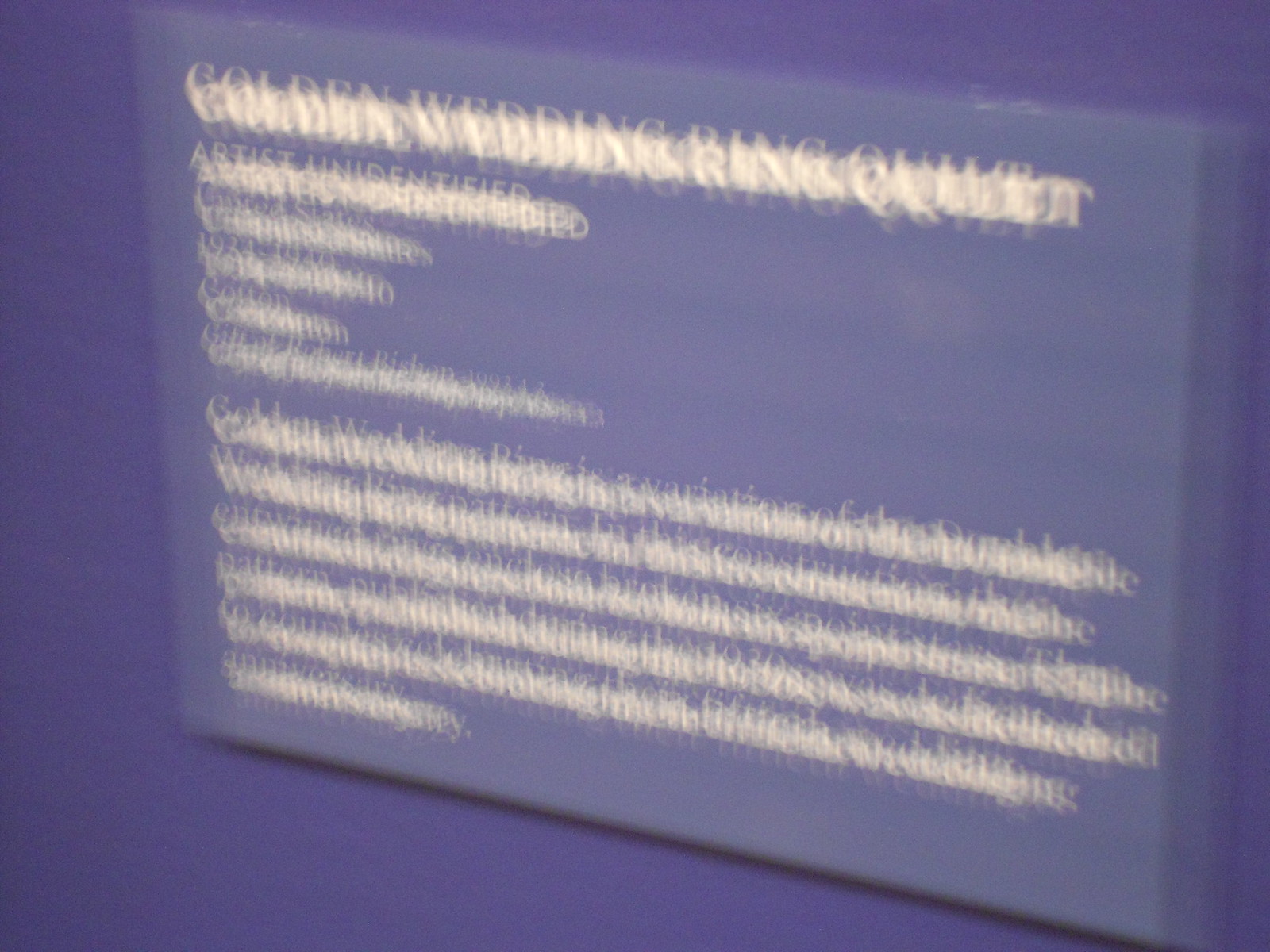The image features a square-shaped, glass-like sign set against a dark purple wall. The sign itself is a lighter shade of purple, creating a subtle contrast with the background. Due to the blurriness of the image, the text is mostly unreadable, but a few significant details can be discerned. At the top, the sign reads "Golden Wedding Ring Quilt," followed by "Artist Unidentified." There appears to be a date range from 1934 to 1940 beneath that. The sign, which is slightly slanted with the left side positioned further back than the right, contains a considerable amount of white text that is mostly illegible due to motion blur. Despite its vivid yet harmonious color scheme, the sign's details remain elusive due to the blurry capture of the image.